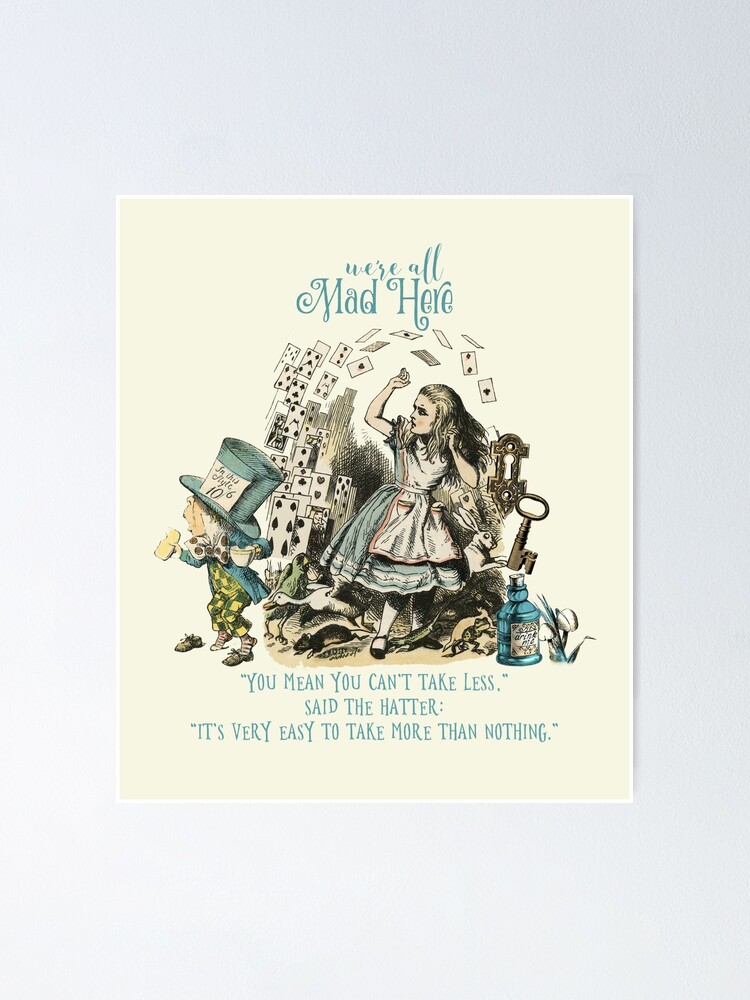This vibrant, whimsical poster depicts a scene inspired by "Alice in Wonderland." At the top, the caption reads, "We're all mad here," setting the theme for the chaotic and fantastical elements within the image. On the left side, the Mad Hatter is portrayed in his characteristic eccentricity, seemingly dancing or moving exuberantly amid flying playing cards. Prominently displayed near him is his iconic hat, marked with "10/6."

Alice stands on the right, dressed in her familiar white and green dress, looking towards the left of the image where the Mad Hatter is. Both characters are surrounded by a variety of chaotic elements, including a swirling collection of poker cards, a key, and a blue bottle labeled "Drink Me." There's also a tea set that the Mad Hatter seems to be handling, adding to the tea party theme from the story.

In the background and around the characters, various whimsical creatures such as a frog, a mouse, a goose, a swan, and some other birds enhance the fantastical atmosphere. A rabbit is also visible behind Alice, evoking the White Rabbit from the tale.

At the bottom of the image, another caption reads, "You mean you can't take less? said the Hatter. It's very easy to take more than nothing," further emphasizing the Mad Hatter's nonsensical wisdom. The overall composition of the poster captures the essence of the "Alice in Wonderland" theme, filled with whimsy, madness, and an array of intriguing details.